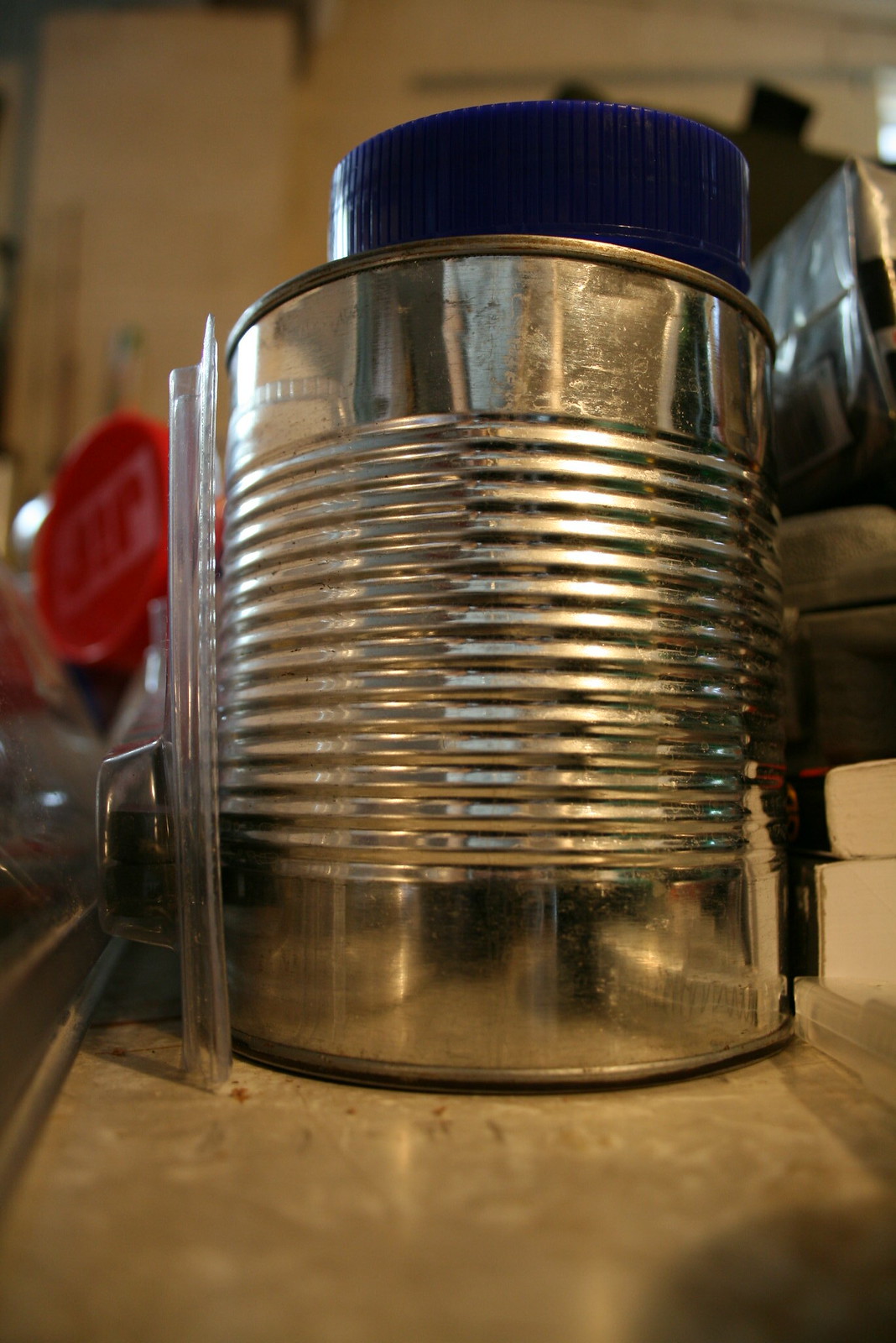In this close-up image, an unlabelled tin can is prominently positioned on a surface that might be a table or counter, though the exact nature of the surface isn't clear. To the left of the can, there is a small plastic straw-like object and a metallic button. Inside the tin can, a blue, thick-lidded jar is visible, though only the lid is distinctly seen. The background of the image features a predominantly beige color scheme with assorted elements, including items in bags and boxes, which are somewhat indistinguishable. Notably, there is also a lid, possibly from a Jif peanut butter jar, lying on its side and slanting to the left.